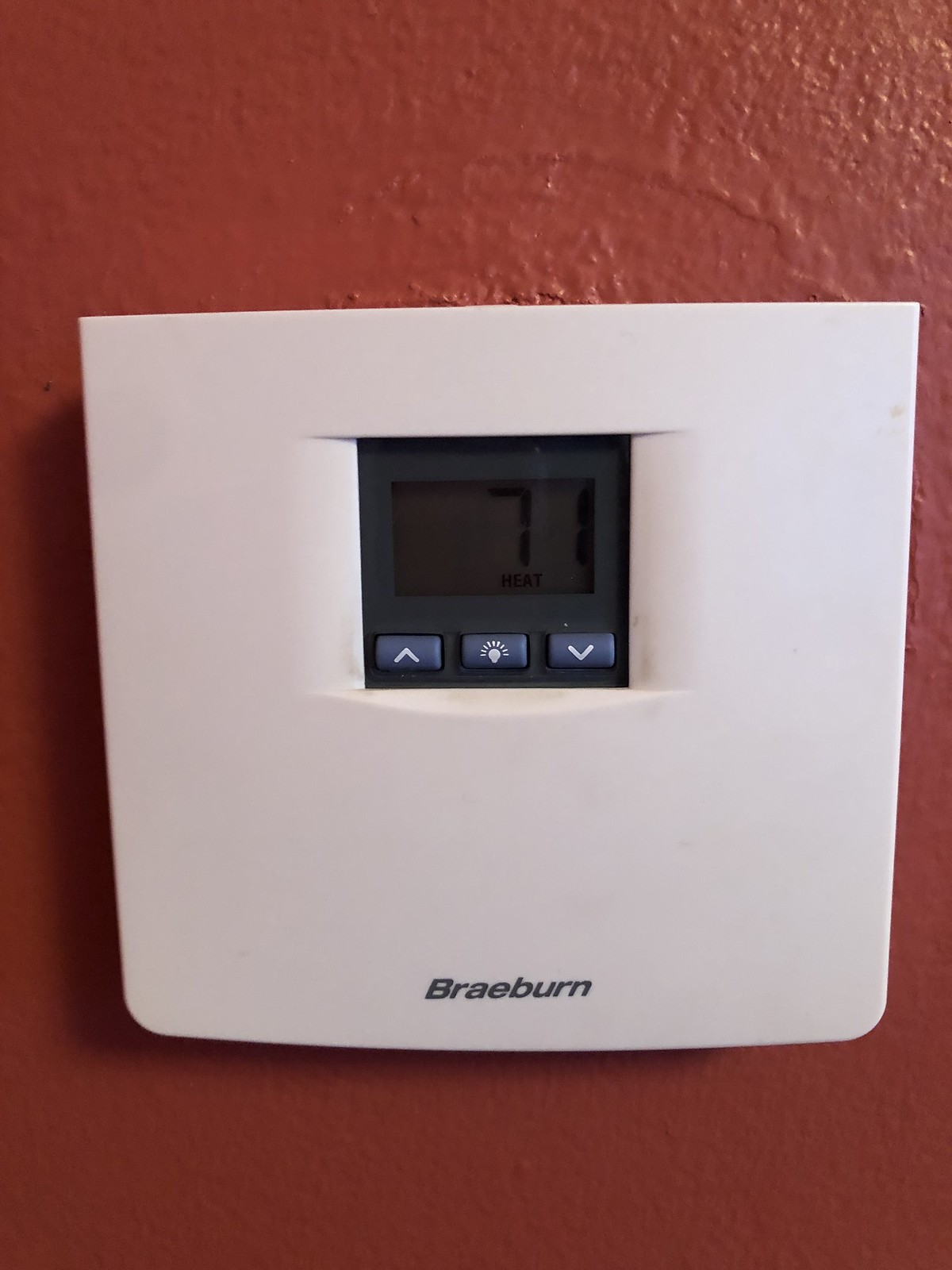This indoor photograph captures a red painted wall adorned with a white Braeburn thermostat. The name "Braeburn" is elegantly printed in gray letters towards the lower center of the device. Dominating the middle of the thermostat is an LCD digital display that reads "71" in black digits, alongside the word "heat." Below the display, three gray adjustment buttons align horizontally: the leftmost button features a white arrow pointing up to increase the temperature, the middle button is marked with a light bulb icon to illuminate the display, and the rightmost button has a downward-pointing white arrow for decreasing the temperature. The sleek design and clear labeling make the thermostat user-friendly and visually appealing against the bold red backdrop.